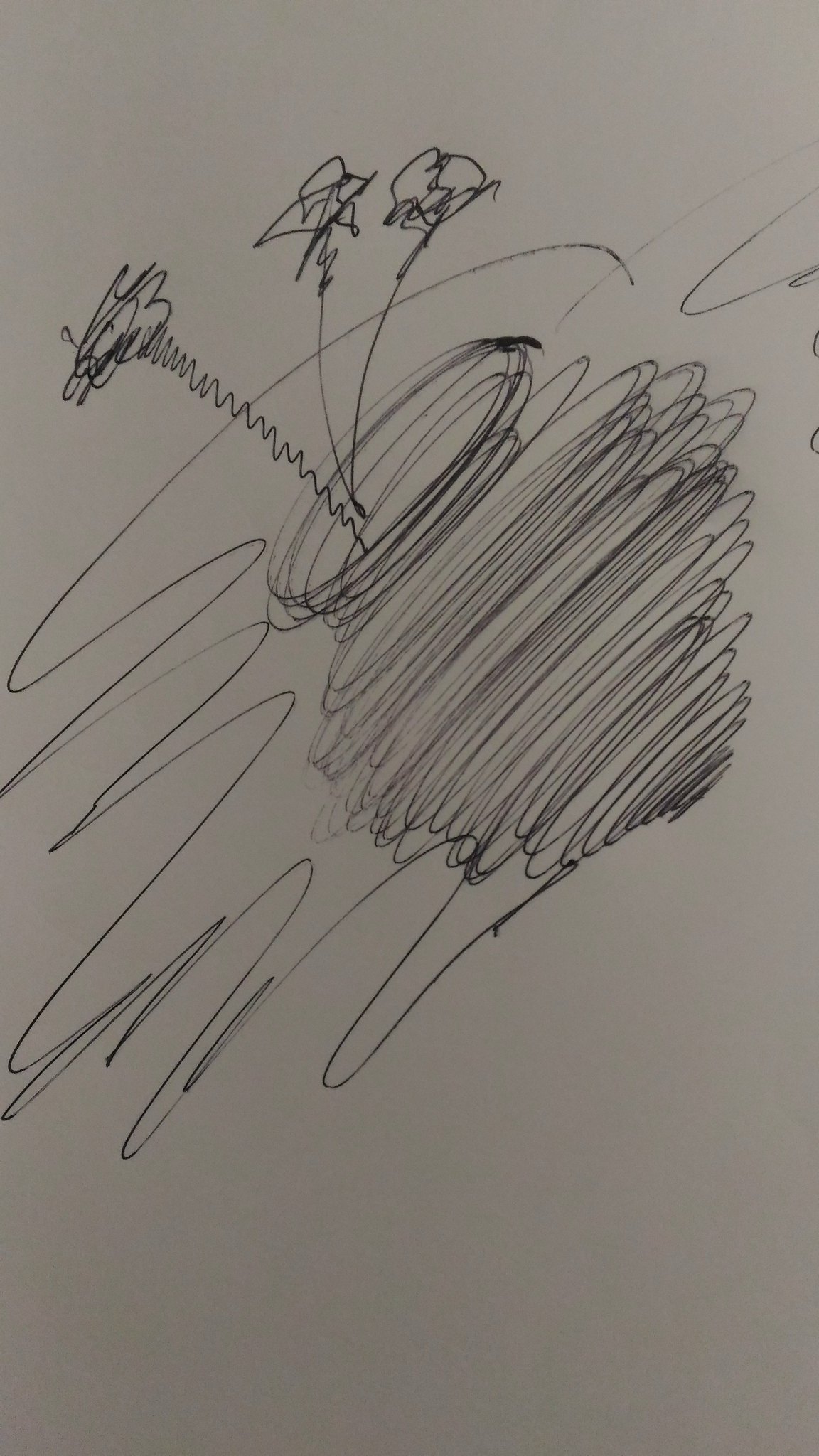In this dimly lit photograph, we see a free-hand pen drawing on a plain sheet of white printer paper. The image is somewhat dark due to suboptimal lighting. The drawing features an abstract, tornado-like vase created from a multitude of circular, swirling lines that give it a dynamic and somewhat chaotic appearance. Emerging from the bottom of the vase, a prominent squiggly line ascends along its left side before curving off to the right, suggesting that the drawing extends beyond the visible frame.

Within the vase, there are three distinct flowers. The flower on the far left has a squiggly line as its stem, while the other two flowers sport curved stems bending to the right. The flowers themselves are composed of loose, scribbled lines that form an impressionistic representation of petals, capturing the essence of flowers without detailed structures. The overall effect is an intriguing blend of abstract artistry and recognizable forms.